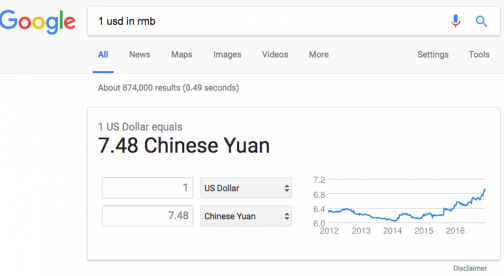The image depicts a Google search results page for the query "1 USD in RMB." At the top of the page, the user has the option to switch between various search categories such as All, News, Maps, Images, Videos, and More. On the right side, settings and tools icons are visible. According to the search results, there are about 874,000 links available, generated in 0.49 seconds.

Centered on the page is a currency conversion widget displaying the exchange rate. It shows that 1 USD equals 7.48 Chinese Yuan (CNY) in larger, bold print. The user interface allows for direct input to convert other amounts and shows a 1 USD value in the top field labeled "US Dollar." The corresponding conversion of 7.48 CNY is displayed in the bottom field labeled "Chinese Yuan."

To the right of the conversion inputs, there is a line graph displaying the exchange rate trend over time, illustrating a recent upward movement in value.